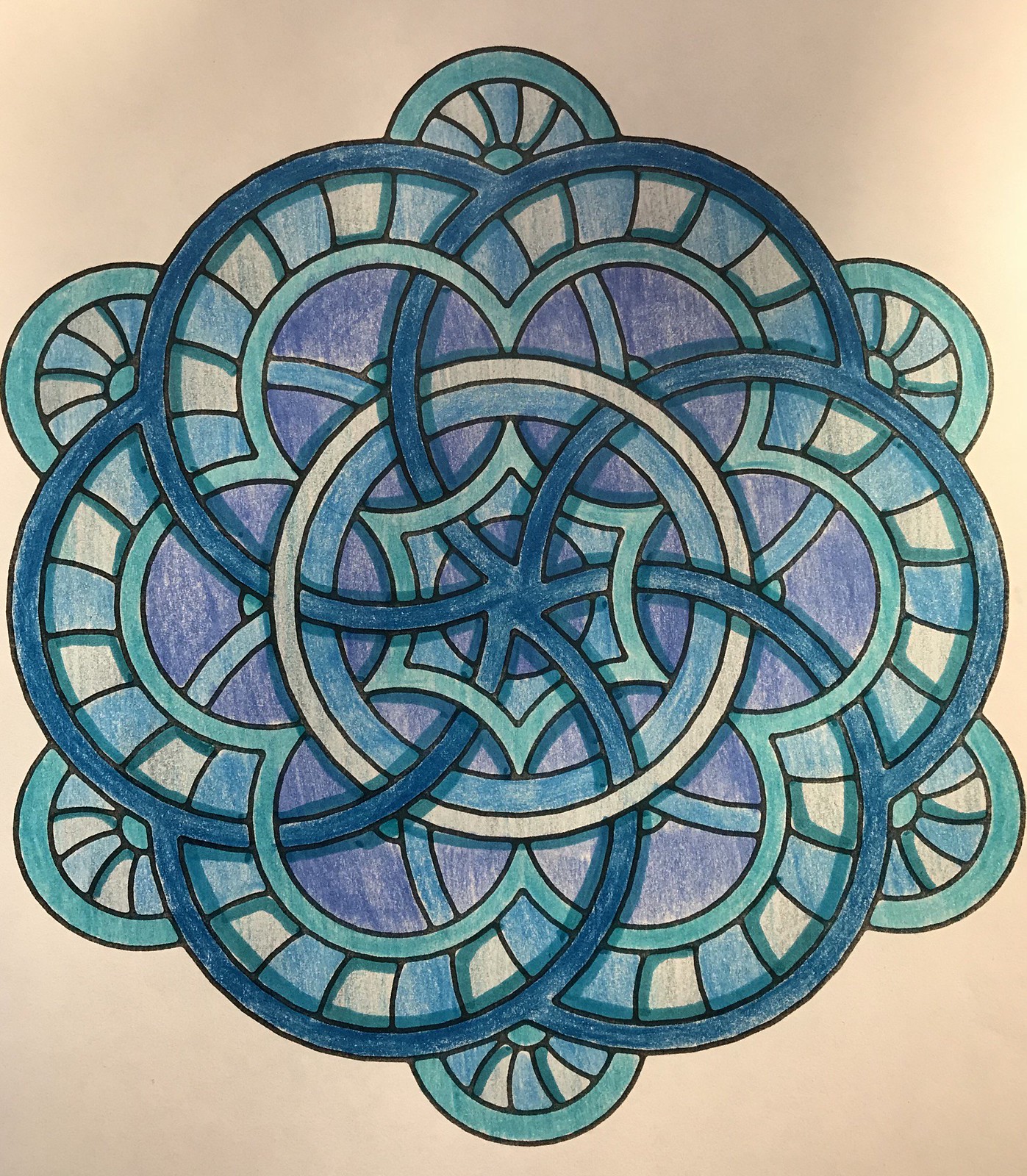The image depicts an intricately detailed drawing, likely created using colored pencils or crayons, possibly enhanced with markers for added depth and shadows. The central focus of the artwork consists of numerous interconnected circles, resembling gears or Celtic designs, which collectively form a complex and mesmerizing pattern similar to that seen through a kaleidoscope. The circles intersect and spiral into each other, with many featuring cut-out designs reminiscent of old-fashioned wheel covers. The color palette includes teal, turquoise, blues, purples, and light plum, all set against a beige background that fades to darker gray at the corners. Notably, one ring in the middle remains uncolored, starkly white, creating a visual focal point amidst the intertwining and overlapping vibrant designs.